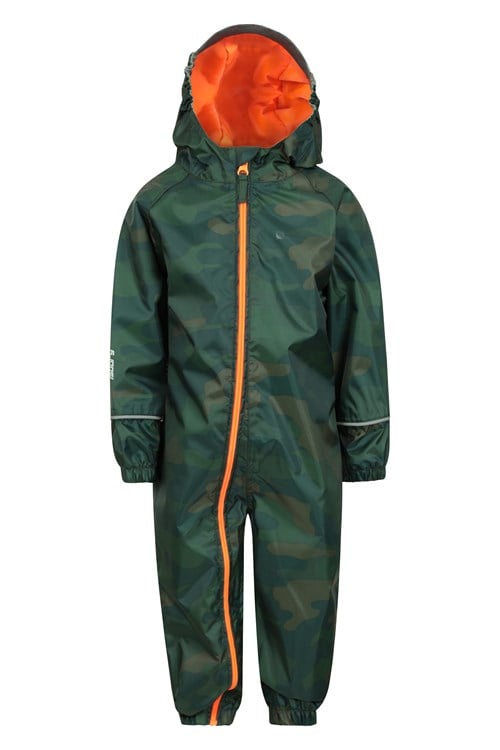This image, likely featured on a children's retail website, showcases a one-piece rain suit designed for kids. The suit's fabric sports a subtle camouflage pattern in shades of dark green, brown, and lighter variations of green, accented by a gray trim. The most striking feature is the vibrant orange zipper that starts at the neckline, runs down the center of the torso, and veers off down the left pant leg, extending to the bottom. This same bright orange color lines the inside of the hood, reminiscent of safety vests worn in the woods to ensure visibility. The camouflage print covers the entirety of the suit, including the hoodie. Additionally, there appears to be some text written on the left-hand side sleeve, though the content is not specified. The suit, resembling a snowsuit or rain suit, is intended to provide both functionality and style for young children. The background of the image is pure white, ensuring that all focus remains on the detailed design of the suit.